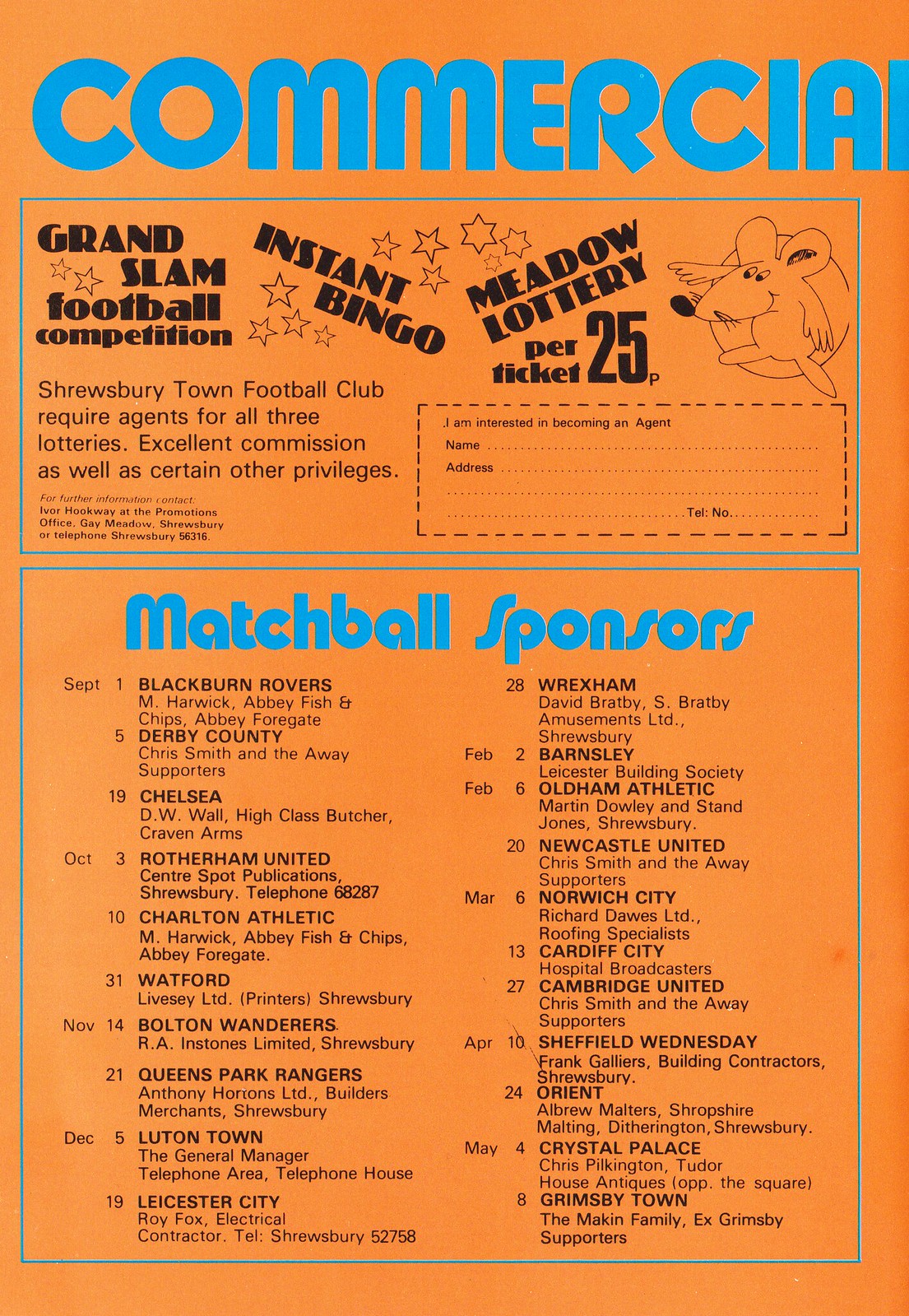The image appears to be a scan from a printed page, possibly from a magazine, with some blue spot color on an orange background. The top section features a bold blue headline partially reading "Commercial," which seems to be slightly cut off. Below this, within a blue rectangular box, is text announcing the "Grand Slam Football Competition Instant Bingo Meadow Lottery" with tickets priced at 25 pence each. Adjacent to this is a blank form where one can fill out their name, address, and telephone number, expressing interest in becoming an agent. To the right of these elements is a sketch of a mouse extending its arm.

The lower portion of the image is framed by a blue outline, with the heading "Match Ball Sponsors" in bold blue letters. This section contains a detailed list of football matches, featuring different teams sponsoring the matches on specific dates ranging from September through May. Listed teams include Blackburn Rovers on September 1st, Derby County on September 5th, Chelsea on September 19th, and Grimsby Town on May 8th among others. The content seems to be styled in the manner of a print publication.